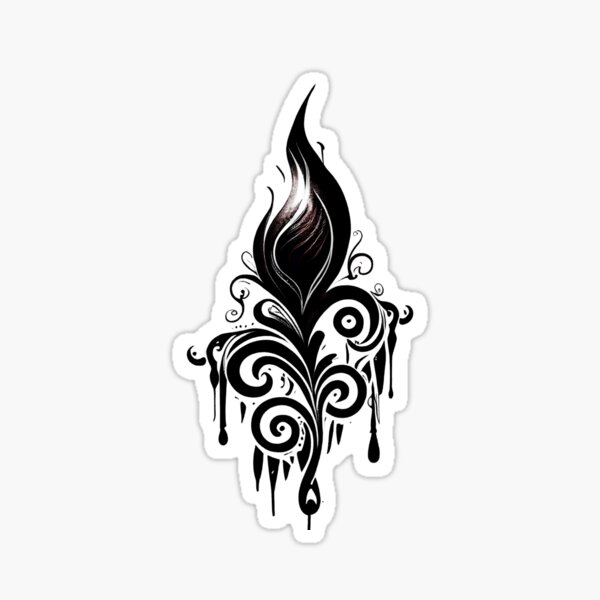This detailed illustration depicts an intricate, black ink drawing on a white background, resembling a flame or a melting candle. The central element is a large, vivid, flame-like shape with ornate swirls and curlicues beneath it, giving an impression of dripping wax or melting matter. Additional elaborate, curling tendrils and spiral patterns extend beneath the main flame, creating an almost floral appearance. The design is highly detailed, featuring numerous tiny dots that add to its ornate quality. The white background mirrors the shape of the illustration, giving the overall image the look of a cutout or sticker, suggesting that it could be printed and used as decorative art.